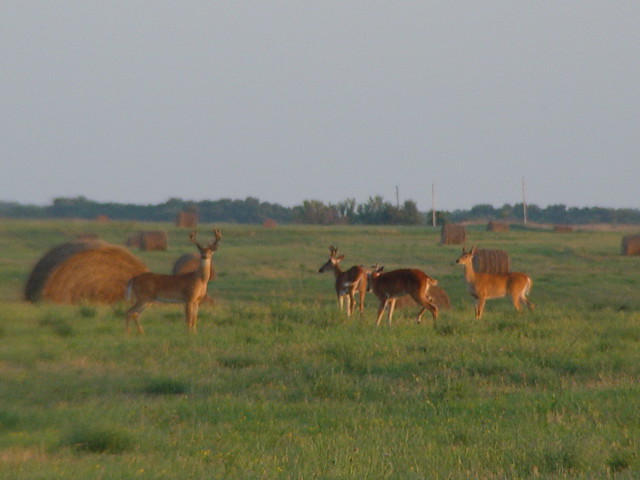The photograph captures an outdoor scene on a later, somewhat overcast day. The sky, a light gray expanse, occupies the upper two-thirds of the image, with no visible clouds. A blurry tree line stretches horizontally across the center of the image, forming a dark green backdrop. Below this, a flat, green pasture extends to the bottom of the frame, dotted with 8 to 10 cylindrical hay bales lying on their sides. Scattered throughout the field, a group of four or five deer moves around, with their motion contributing to the image's overall blur. One prominent deer on the left, featuring noticeable antlers, stands still and gazes directly at the photographer. The remaining deer, smaller and also brown with white markings, appear less alert as they move through the scene. Additionally, three telephone poles are faintly visible in the background, reinforcing the rural setting.